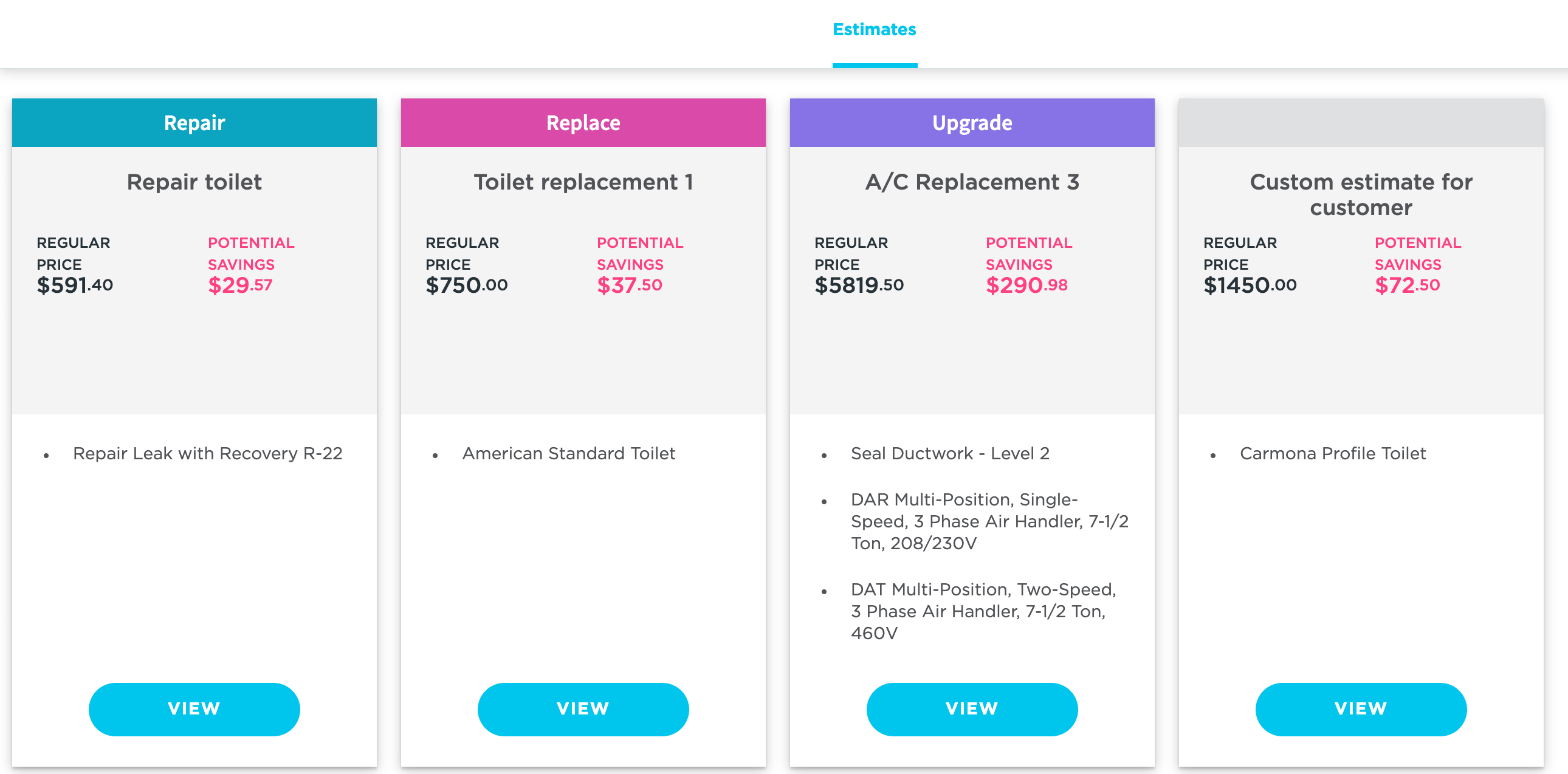This page serves as the signup section for a website offering a variety of services, primarily focusing on HVAC and plumbing, but potentially including other services as well. The layout features vertically-oriented rectangles, each distinguished by a colored banner at the top that titles the respective service category.

1. **Repair** - Light blue banner.
2. **Replace** - Purple banner.
3. **Upgrade** - Dark bluish-purple banner.
4. **Custom Estimate** - Grayed out area with no specific title, labeled underneath as "Custom Estimate for Customer."

Below these banners, the individual services are listed from left to right:

1. **Repair Toilet**
2. **Toilet Replacement One**
3. **AC Replacement Three**
4. **Custom Estimate for Customer**

For each service, there is detailed pricing information, highlighting the regular price and potential savings in a distinct reddish-pink color. Following this, each section contains a bulleted list on a white background with specific service details, such as:

- Repair leak with recovery $122
- Sealed ductwork level 2
- Carmona profile toilet

At the very bottom of each service section, there is a light blue button with "View" written in white text, allowing users to get more information.